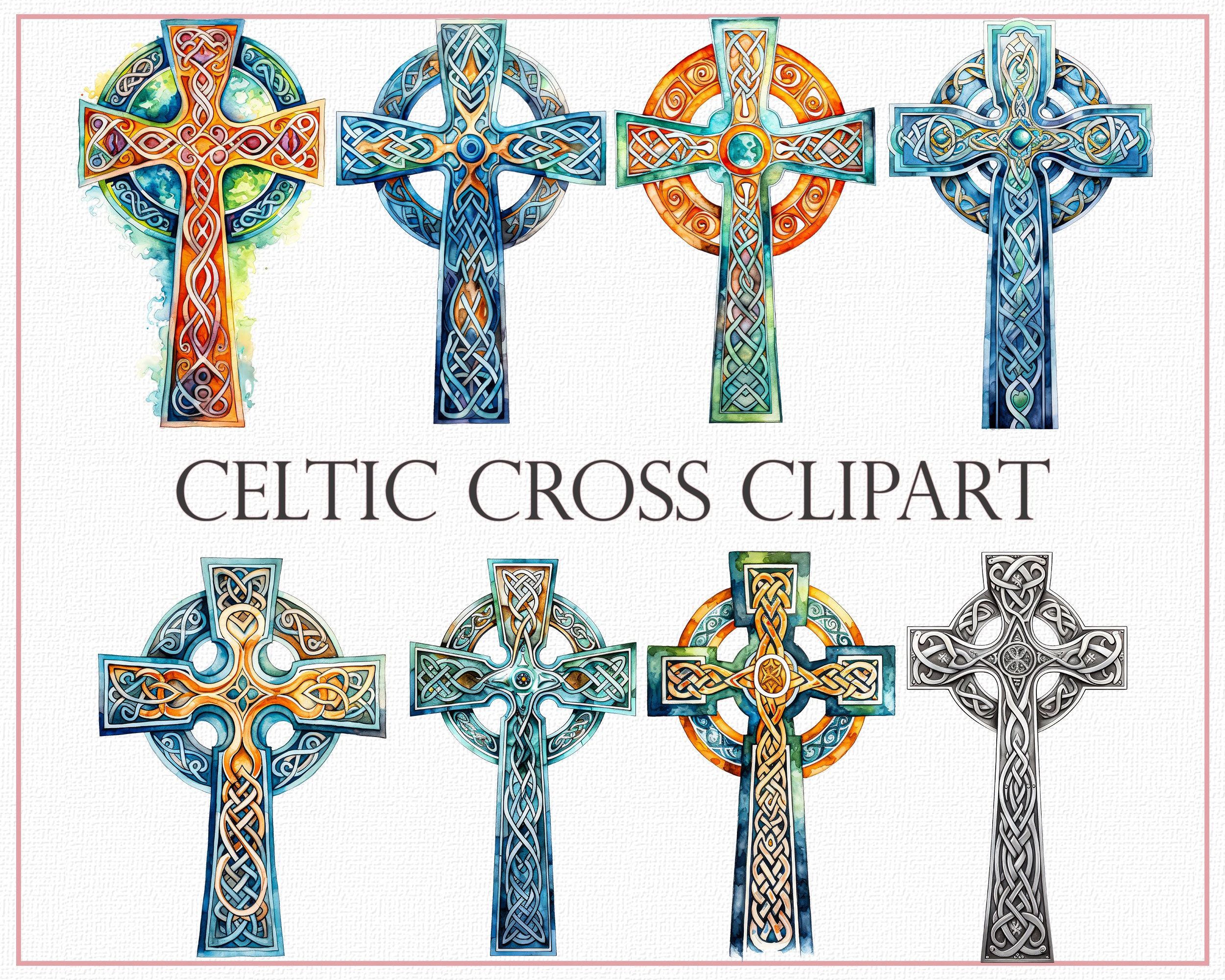This is a large image with a thin, rose-colored border around it and a white background. The image features eight distinctive Celtic crosses, arranged in two rows with four crosses in each row. In the center of the image, in all-caps dark gray letters, it reads "CELTIC CROSS CLIP ART."

In the top row, each cross has a circle behind the T-shaped top and varies in color and design:
1. The first cross is predominantly orange, blue, and yellow.
2. The second cross is mostly blue and brown.
3. The third cross features an orange circle behind a mainly green cross.
4. The fourth cross is primarily blue with a touch of gold.

In the bottom row, the designs continue with a mix of hues:
1. The first cross combines gold and blue.
2. The second is a blend of gray and gold or brown.
3. The third cross showcases orange, blue, and green.
4. The fourth and final cross in the lower right corner is gray, giving a metallic appearance.

This thoughtfully arranged image is likely designed for a website, serving as a detailed collection of Celtic cross clip art.